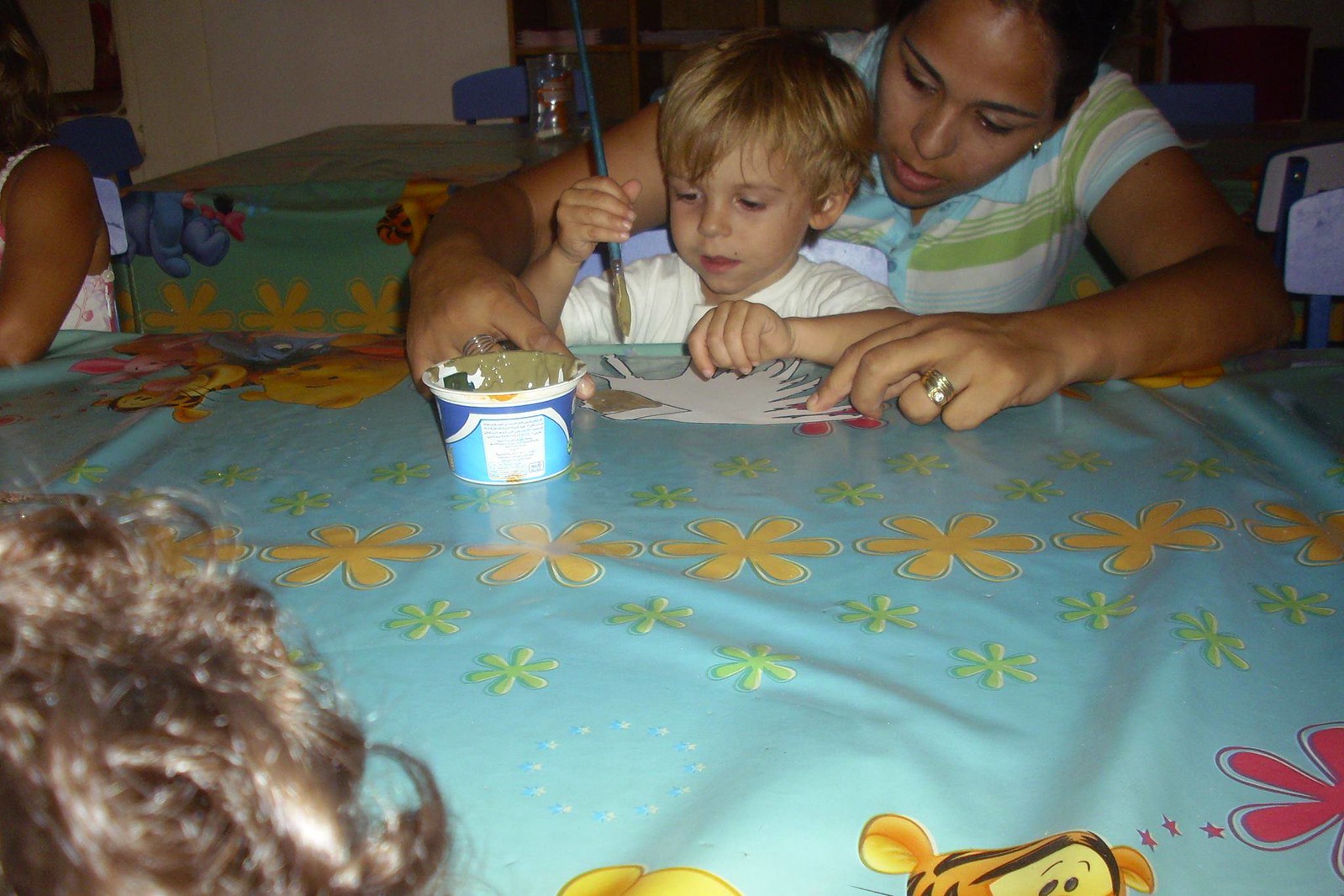In the upper right-hand corner of the image, a dark-complected woman with black hair pulled back, likely the mother, is seated behind a young blonde-haired child, probably around three years old. The mother, wearing a white short-sleeved shirt with green and blue stripes, is guiding the child as he engages in an arts and crafts project. The boy, dressed in a white shirt, holds a blue-handled paintbrush with a light green paint in his right hand, applying it to a piece of paper in front of him. 

There's a light blue tablecloth adorned with light yellow and light green flowers, and a partial view of the character Tigger from Winnie the Pooh is visible at the bottom of the image. The scene is dark, likely due to the use of a flash, giving it a dim ambiance. In the background, a second table can be seen, adding depth to the setting. Additional figures are partially visible: another child's hair in the upper left-hand corner and an undefined person in the lower left-hand corner of the picture. The photo captures a shared moment filled with creativity and familial bonding.